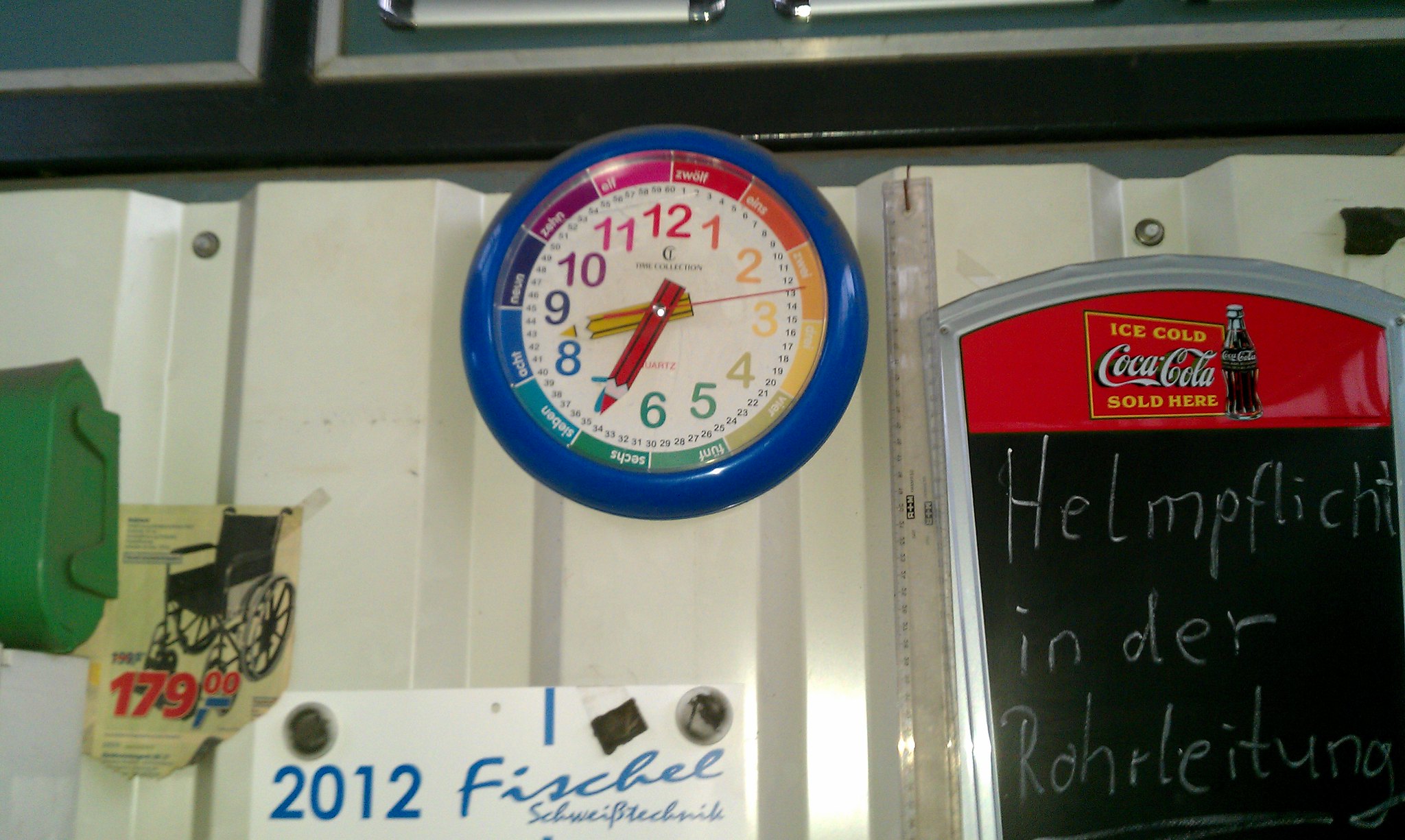The image depicts a section of a wall in what appears to be a German cafe or roadside stop. The wall itself is composed of cream or light silver corrugated metal panels, bolted together in small sections with crimped edges. Dominating the wall is a chalkboard adorned with a vintage Coca-Cola advertisement featuring a red logo that reads "Ice Cold Coca-Cola, Sold Here" and a cartoon-style bottle of Coca-Cola beneath it. There's German writing on the blackboard stating, "Helm Pflicht in der Ruhr-Hotel," alongside the year "2012" and the term "FISCHLSCHWEIFTECHNIK."

Adjacent to the blackboard is a colorful child's clock with a royal blue frame. The clock is designed for learning, prominently displaying rainbow-colored numbers. Further to the left, there is a green container mounted on the wall, likely a paper towel dispenser. Nearby, a newspaper advertisement for a wheelchair priced at £179.99 is cut out and affixed to the wall with tape. Just the edge of a first aid box can also be seen in the image. Adding to the eclectic array of items, there is a piece of paper displaying a wheelchair and the price “179” in red font, and a white sign with the year "2012" and the partial text "FISCHL.” Above the wall, black trim runs horizontally across the top of the picture, completing the detailed and varied scene.